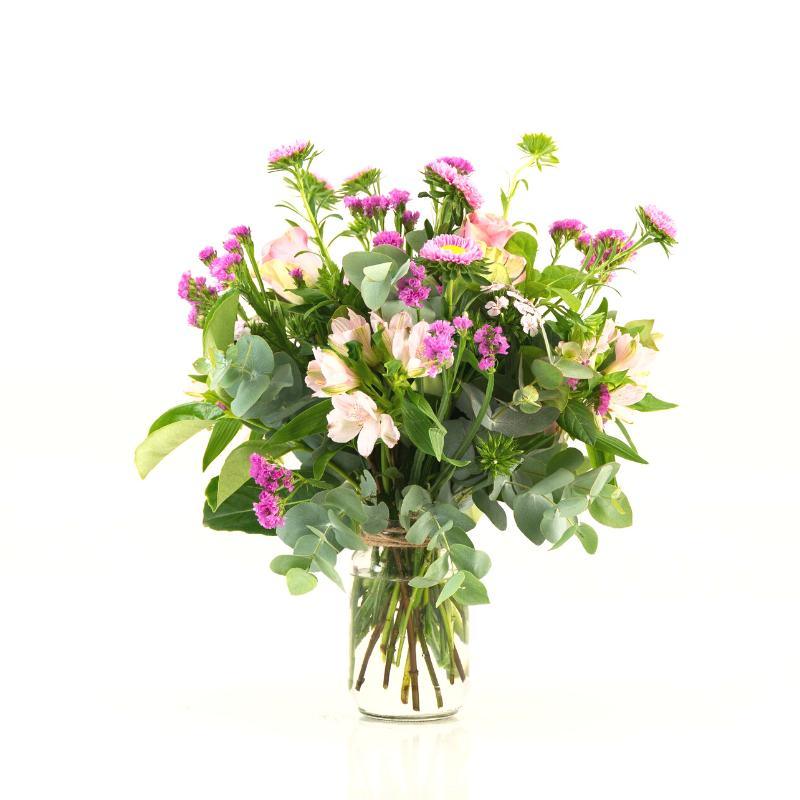This image depicts an elegant bouquet arranged in a cylindrical clear glass vase filled with water, accentuated by a piece of twine wrapped around the vase's neck. Set against a plain white background, typically used for product images on a florist's website, the assortment features a delightful mix of flowers and greenery. Visible through the glass are the stems submerged in water. The bouquet comprises a variety of flowers including large, flat white blooms with broad petals, clusters of small purple and white flowers, and vibrant pink and yellow flowers. Mixed among the flowers are stems with diverse leaf shapes, ranging from round to oval and teardrop. The arrangement exudes a fresh, lush appearance with an abundance of green foliage giving it volume and texture. The overall presentation is both charming and carefully curated, making it an appealing floral display suitable for any occasion.